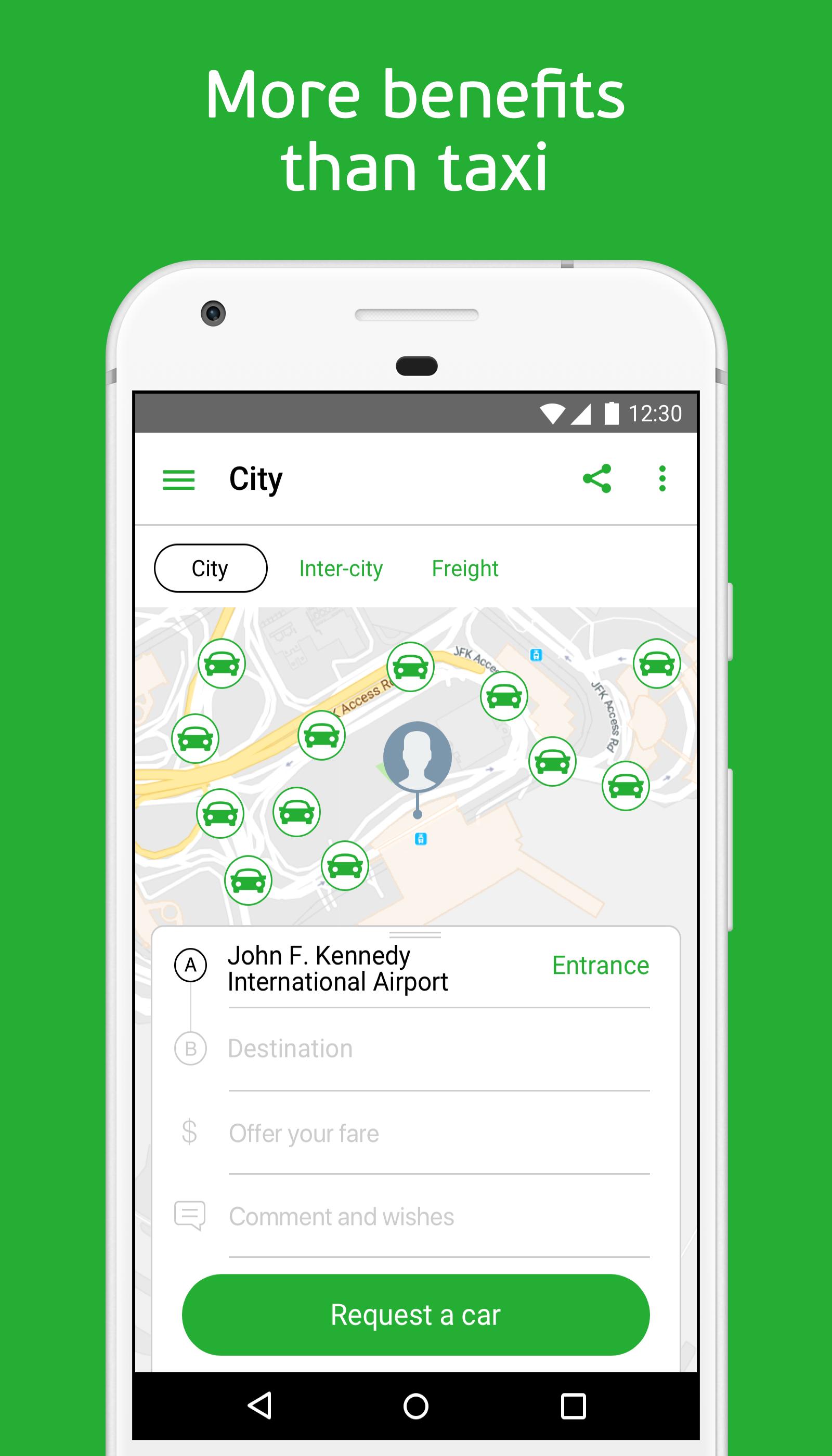The advertisement image promotes a car service through a green vertical rectangle. At the top, bold white text reads: "More benefits than taxi." 

Central to the design is an overlay of an iPhone screen. The top-right corner of the iPhone displays typical status indicators: a strong Wi-Fi signal, full cellular reception, a nearly full battery, and the time "12:30". Beneath these, the phone's interface shows the word "City".

The lower part of the phone screen features three tabs, with the "City" tab highlighted, followed by "Intercity" and "Freight". Below these, a map is dotted with 12 white circles containing green car icons. A larger circle with a person's head icon marks a specific location. This point is in proximity to labelled streets including "JFK Access Road" and another partially visible "Access Road".

Highlighted below the map, the text reads: "A. John F. Kennedy International Airport entrance." In lighter text beneath, it states: "B. Destination," "Dollar sign, offer your fare," and "Comments and wishes." At the bottom of the page, a prominent button says, "Request a car."